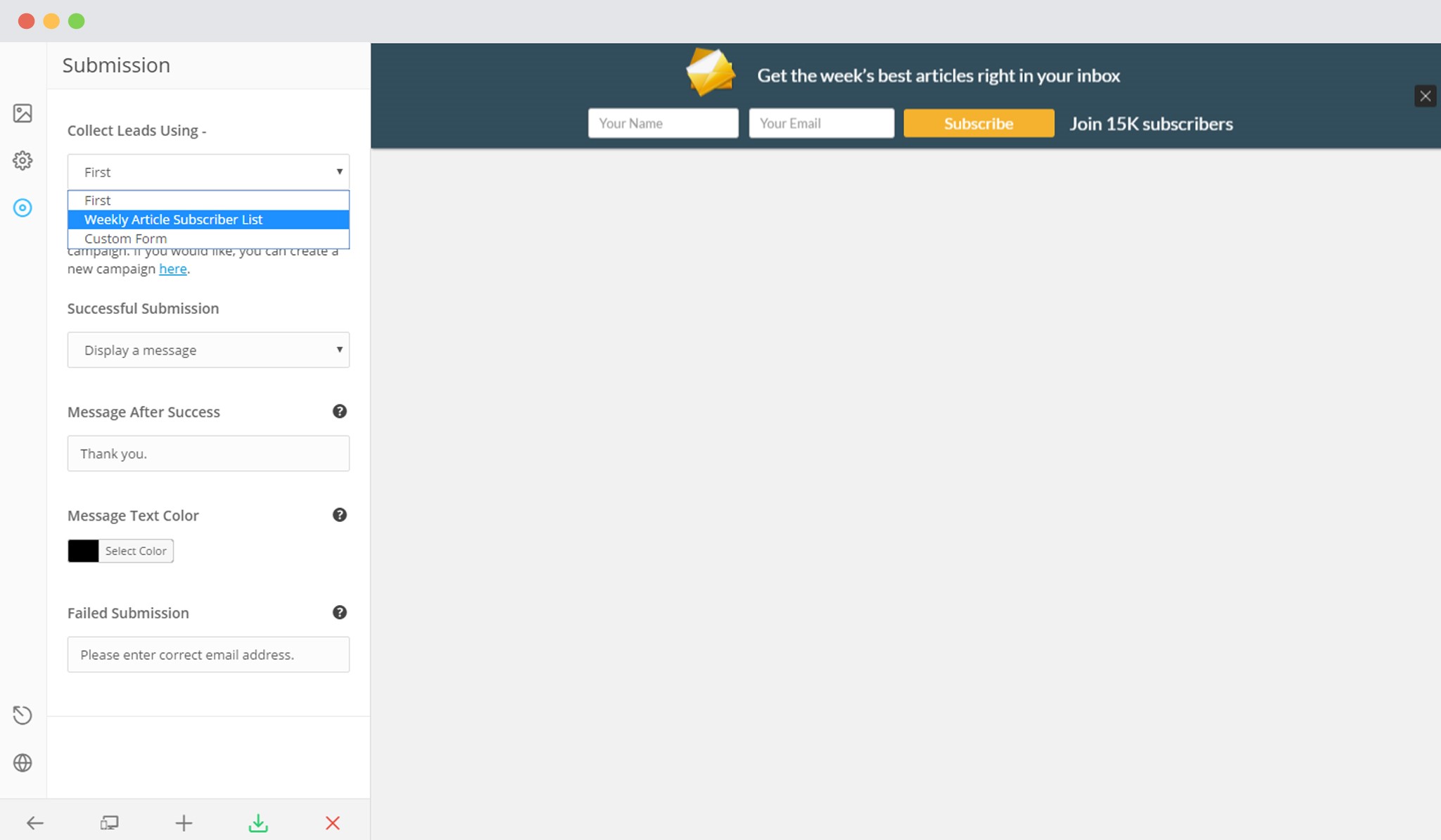The image depicts a structured user interface component within a gray rectangle extending across the top of the screen. In the upper left corner, three small circular buttons are arranged horizontally: a red button, a yellow-orange button, and a green button. Below this, a white vertical rectangle spans the length of the gray rectangle, serving as a column for various labels and instructions.

At the top of this column, the label "Submission" appears in black text. Following this, from top to bottom, a series of phrases are listed:
- "Collect leads using: first, weekly subscription list"
- "Custom form"
- "New campaign"
- "Successful submission: Display a message"
- "Message after success: Thank you, message text color"
- "Failed submission: Please enter correct email address"

To the right of this text, occupying the center to the far-right edge of the image, is a prominent black rectangle with the phrase "Get the week's best articles right in your inbox." Below this, there are two white input fields labeled "Your Name" and "Your Email," followed by an orange button with the word "Subscribe" in white text. Under this button, a smaller text reads "Join 15k subscribers."

The remainder of the column is unoccupied within the gray rectangle. At the very bottom of this column are several icons: an arrow pointing left, a stack of pages, a plus sign, a green arrow pointing downwards into a half rectangle, and a red X.